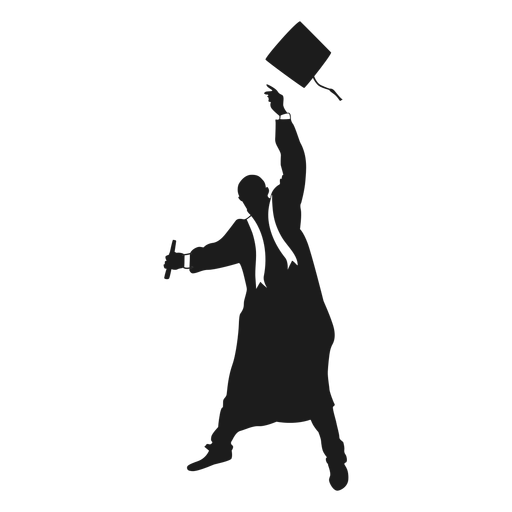This black-and-white clipart image is a detailed digital silhouette of a graduate in full celebration. The illustration shows the person dressed in a traditional black graduation gown, accented by a white sash draped around their neck and hanging down in front. The cuffs of the graduate's shirt are slightly visible, protruding from beneath the sleeves of the gown. 

The graduate’s legs are spread apart, giving a stance of triumph and excitement. The individual is captured in the midst of throwing their graduation cap into the air. The cap, with its distinctive square shape and tassel flowing as if caught mid-throw, hovers just above the celebrant’s outstretched right hand, which reaches towards the sky. In the graduate's left hand, they clutch a rolled-up diploma tightly, signifying their recent achievement. The entire graphic is based on a transparent background, allowing the celebratory scene to stand out prominently.